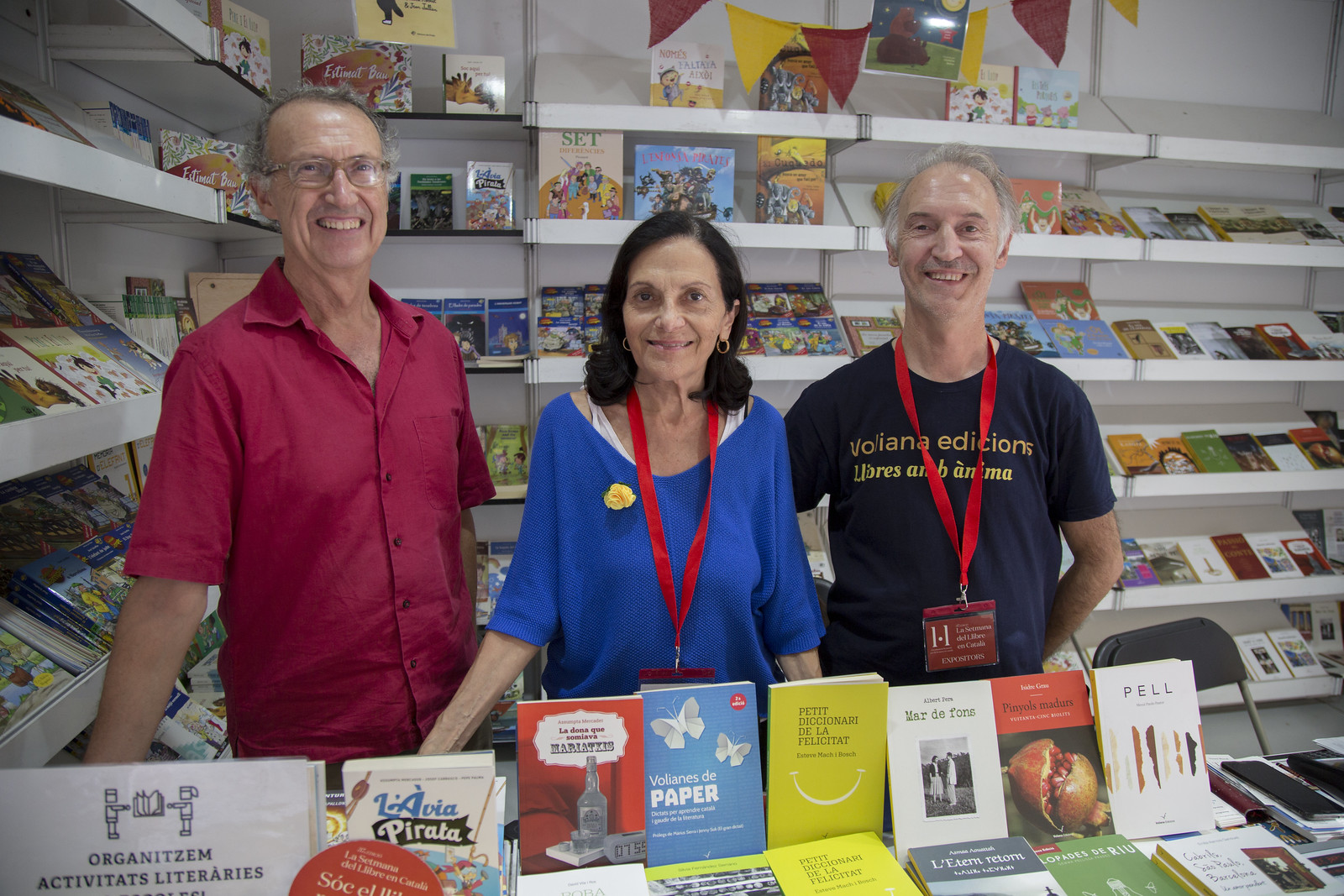The photograph captures a lively scene at what appears to be a bookstore or library during a book fair. Three people, all smiling warmly at the camera, stand behind a table laden with various books, some standing upright and others lying flat. The background features shelves brimming with books and colorful pennant flags in red and yellow, enhancing the festive atmosphere.

On the far left stands an older Caucasian man, wearing a short-sleeved red button-down shirt. He has gray hair, appears to be balding, and wears glasses. His right hand is casually resting on the table, partially obscured by the books.

In the center is an older woman with shoulder-length dark hair parted down the middle. She is dressed in a blue drapey shirt over a white tank top, accessorized with a red lanyard and a yellow flower pinned to her shirt. She also has gold earrings and dark eyes.

To the right stands another older Caucasian man, also gray-haired and balding. He’s sporting a blue short-sleeved T-shirt that reads "Violana Editions Libris and Anima," partially covered by a red lanyard. Like the others, he’s smiling and appears to be enjoying the moment.

The scene warmly captures the essence of a community gathering centered around the love of books.